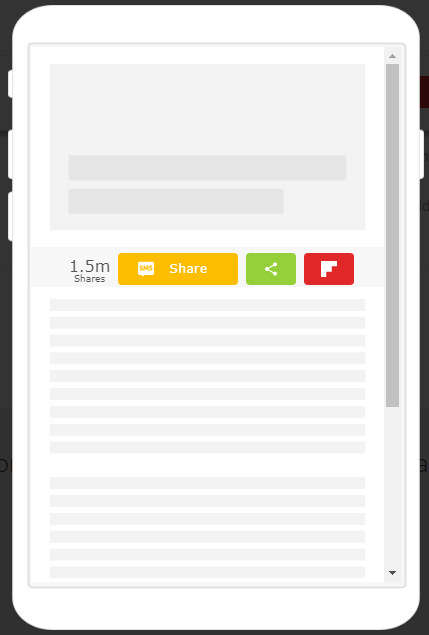The image is a screenshot of a minimalist interface, likely from a social media platform or a related application, showing limited but distinct elements. Dominating the center of the screen is a text indicating "1.5 million shares." To the immediate right, there are three adjacent share buttons, each in different colors: the first is an orange button with white text, the second is a green button with a share icon and white text, and the third is a red button with white text, potentially representing a sharing option related to another social media service. The background of the screenshot is entirely white, giving it a blank and loading appearance, suggesting the site may not have fully loaded. This screenshot could have been captured either on a mobile phone or tablet, based on the interface and design elements visible.